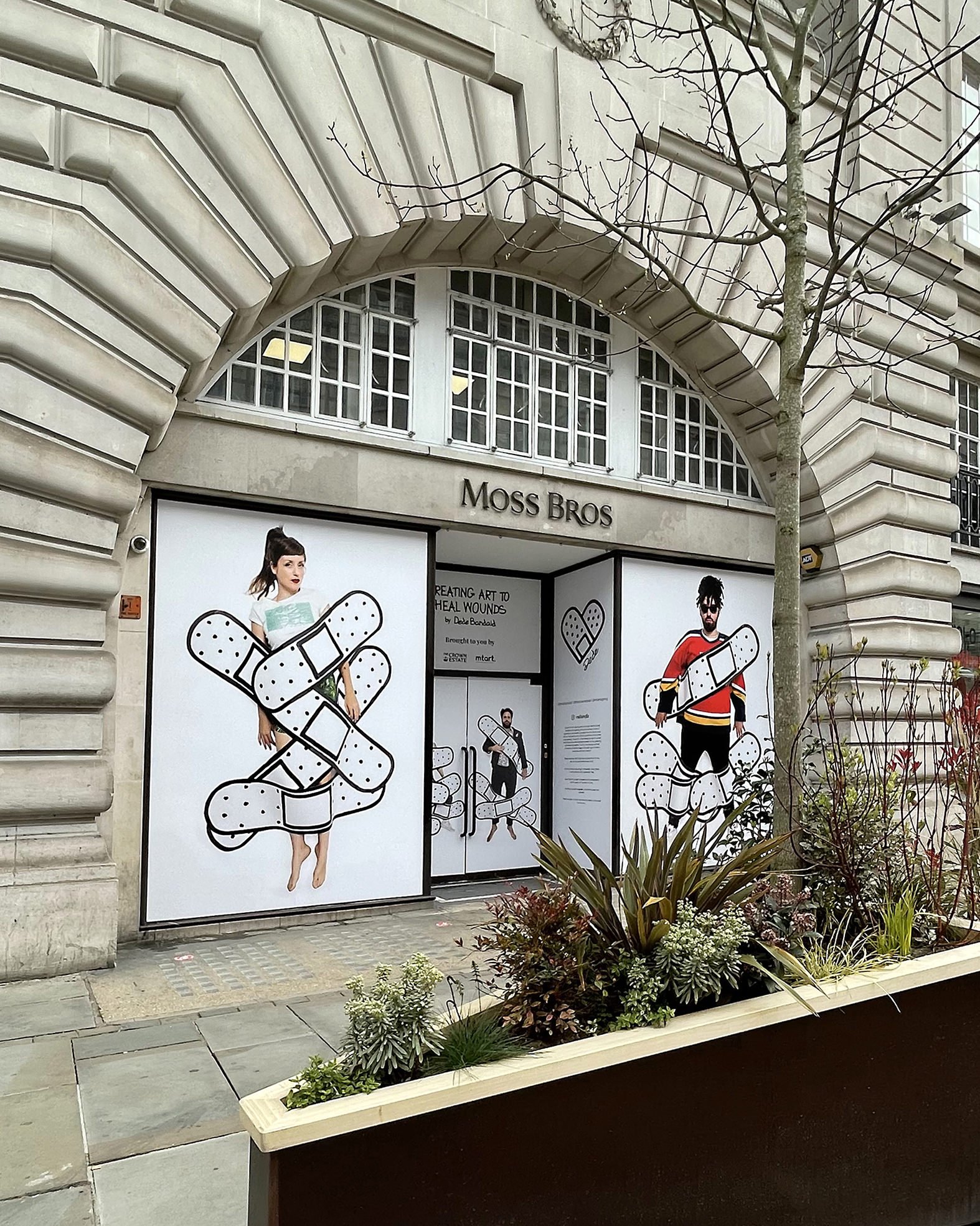This is an exterior photograph of a store named Moss Brothers, captured from the street perspective. The building's entrance is distinguished by a prominent arched doorway adorned with numerous small windows, through which lights inside the building are visible. Below this arch, a black cement sign displays the name "Moss Brothers," leading down to a tiled or concrete sidewalk that features a black and white planter with plants protruding from it. Flanking the entrance door are two striking pieces of artwork on white backgrounds: to the left, an image of a young woman covered in white band-aids over her clothes; to the right, a portrait of a bearded man with sunglasses, similarly adorned with white band-aids over his red shirt and black pants. Additionally, the door itself bears a message about creating art to heal wounds. The building's exterior is constructed of large white stone, giving it a solid and imposing appearance.